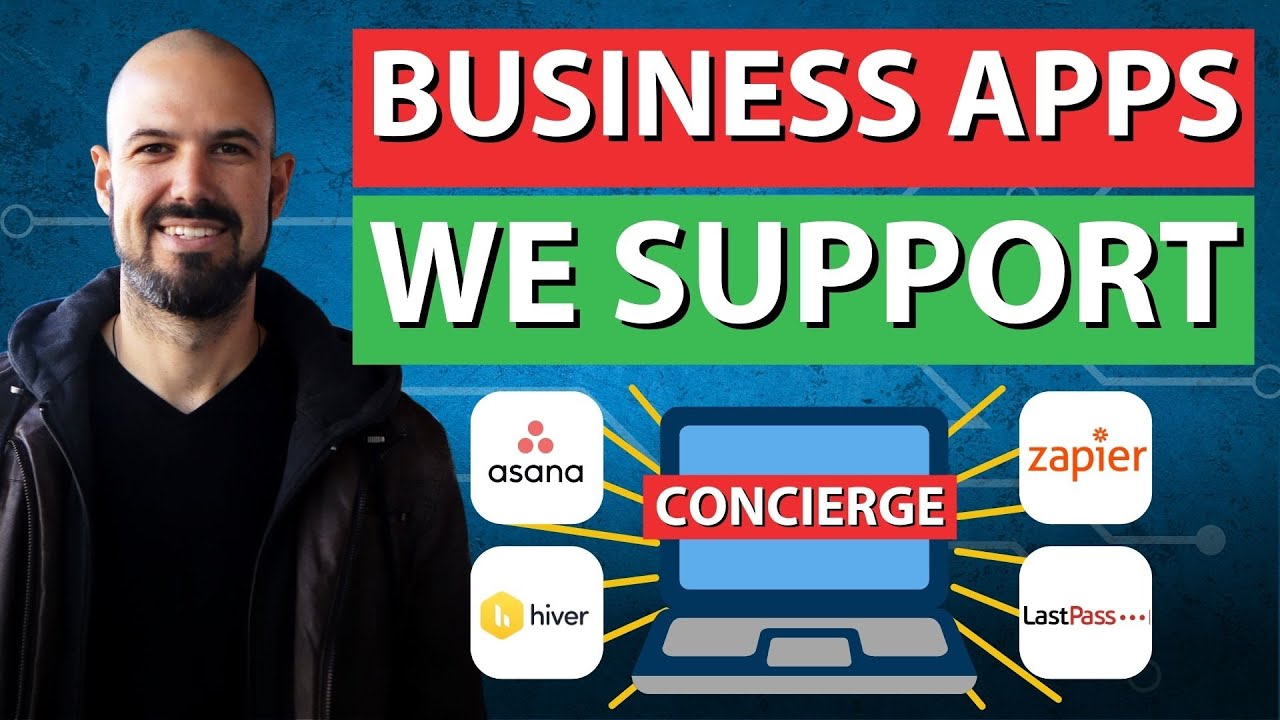This visually engaging graphic appears to be designed for a social media post or website banner. The background features a rich blue hue adorned with a lighter blue circuit board pattern, evoking a tech-savvy and modern aesthetic. On the left side of the image, a photograph of a man is prominently positioned, seamlessly integrated with the tech-themed backdrop. 

At the top right corner, a conspicuous red rectangle boldly announces "Business Apps" in large, white letters, immediately drawing attention. Beneath this, a sizable green box declares "We Support" in similarly large, white text, together forming the message: "Business Apps We Support." 

In the bottom right corner, a clipart illustration of a laptop is centrally placed, with a red box overlaying its screen, emblazoned with the word "Concierge" in striking white letters. Flanking this centerpiece, two white boxes containing logos are positioned to the left of the laptop, with two additional white boxes with logos to its right, creating a coherent and balanced layout.